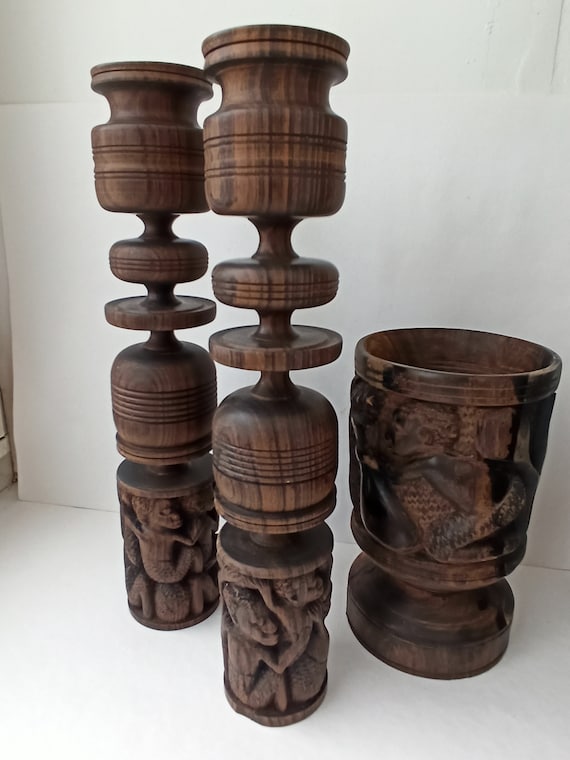This color photograph showcases three exquisitely crafted wooden objects arranged on a pristine white surface against a white backdrop. On the right is a goblet, made of dark-stained wood, featuring intricate hand-carved motifs, including a relief of a man. The goblet has a solid base, a narrow stem, and a beautifully finished rim. To the left are two tall, cylindrical candlesticks, also in dark-stained wood. Each candlestick is adorned with detailed carvings at the base, resembling sculptural depictions of people. The candlesticks are composed of layered disks around a central rod, showcasing various rounded shapes and flaring sections, culminating in a flared top where a candle would sit. The craftsmanship of these pieces highlights a sophisticated combination of woodturning and detailed relief carving, making them remarkable artifacts.